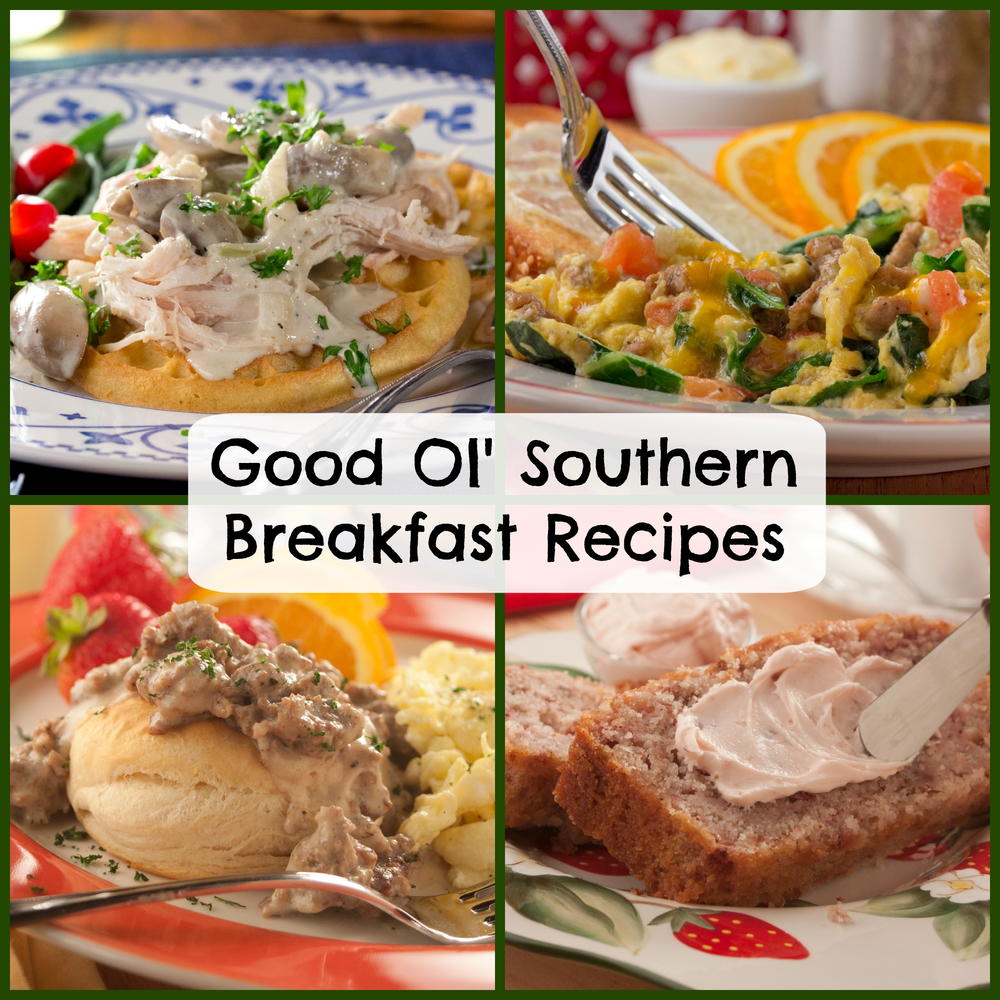This image, resembling a book cover, is a collage of four distinct food photos, each in one quadrant. Central black text on a white background reads "Good Old Southern Breakfast Recipes," with the entire collage outlined in green. In the top left quadrant, there are waffles topped with a mixture of seafood and vegetables. The top right quadrant showcases a plate featuring slices of fresh orange alongside a hearty mix of eggs, sausage, and green peppers. In the bottom left quadrant, there's a plate with biscuits generously covered in creamy sausage gravy, accompanied by strawberries and orange slices. Lastly, the bottom right quadrant shows a knife spreading butter or cheese on a slice of bread.